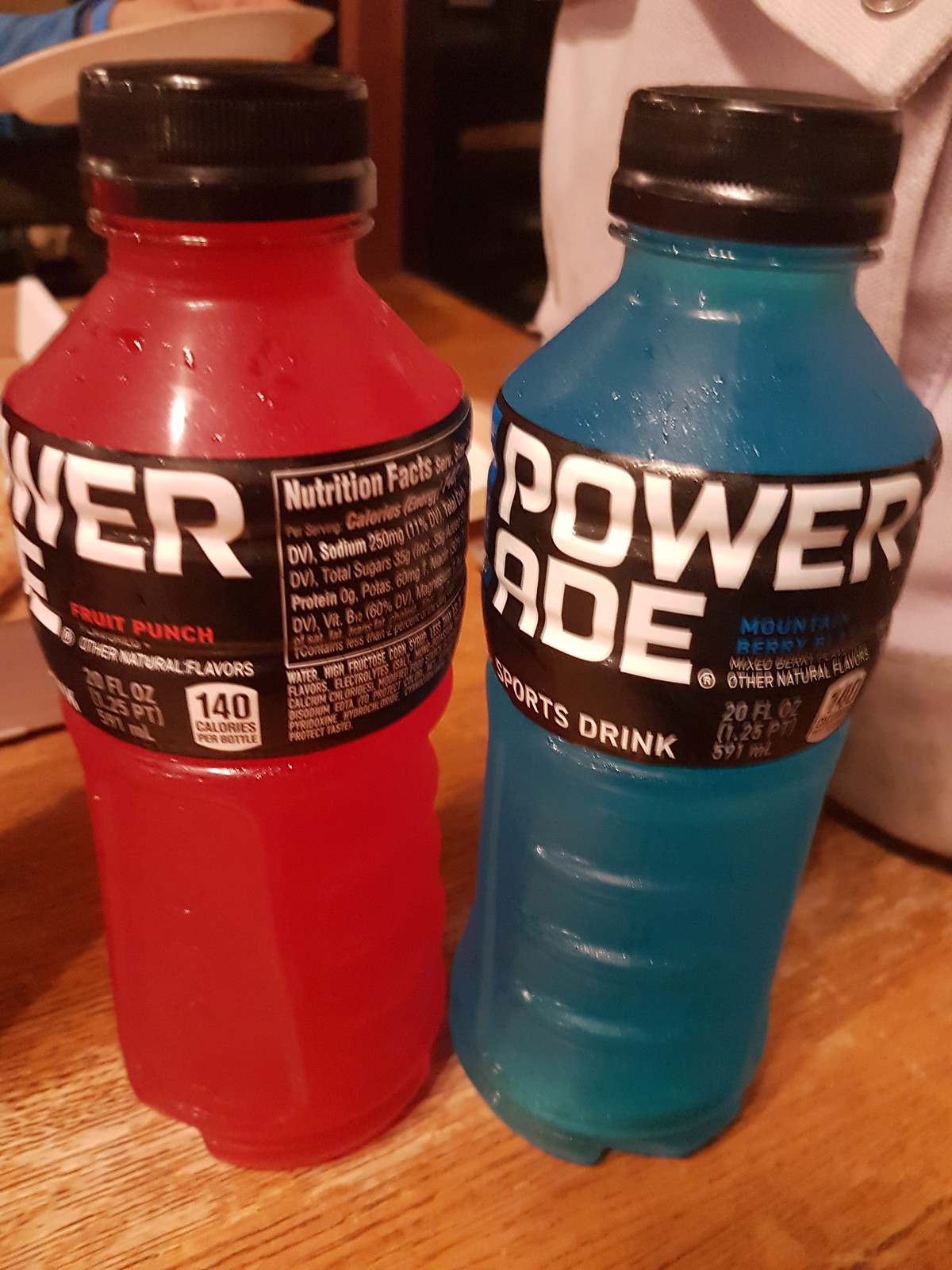In this detailed image, two unopened bottles of Powerade—one Fruit Punch and one Mountain Berry Blast—are positioned side by side on a light brown wooden table, which displays some white scuff marks. The Fruit Punch on the left is a vibrant red, and the Mountain Berry Blast on the right is a bright blue. Each bottle features a distinctive black label with bold white lettering: "Power" at the top and "Ade" at the bottom, sporting the phrase "sports drink." Both bottles are capped with black lids and boast grip-friendly ridges. They exhibit noticeable condensation, suggesting they were recently taken out of the refrigerator. The photo also captures a white cloth or bag positioned next to the blue Powerade bottle on the right. In the background, a person wearing a light blue sweater, visible in the top left corner, appears to be holding a plate, adding a touch of everyday life to the scene.